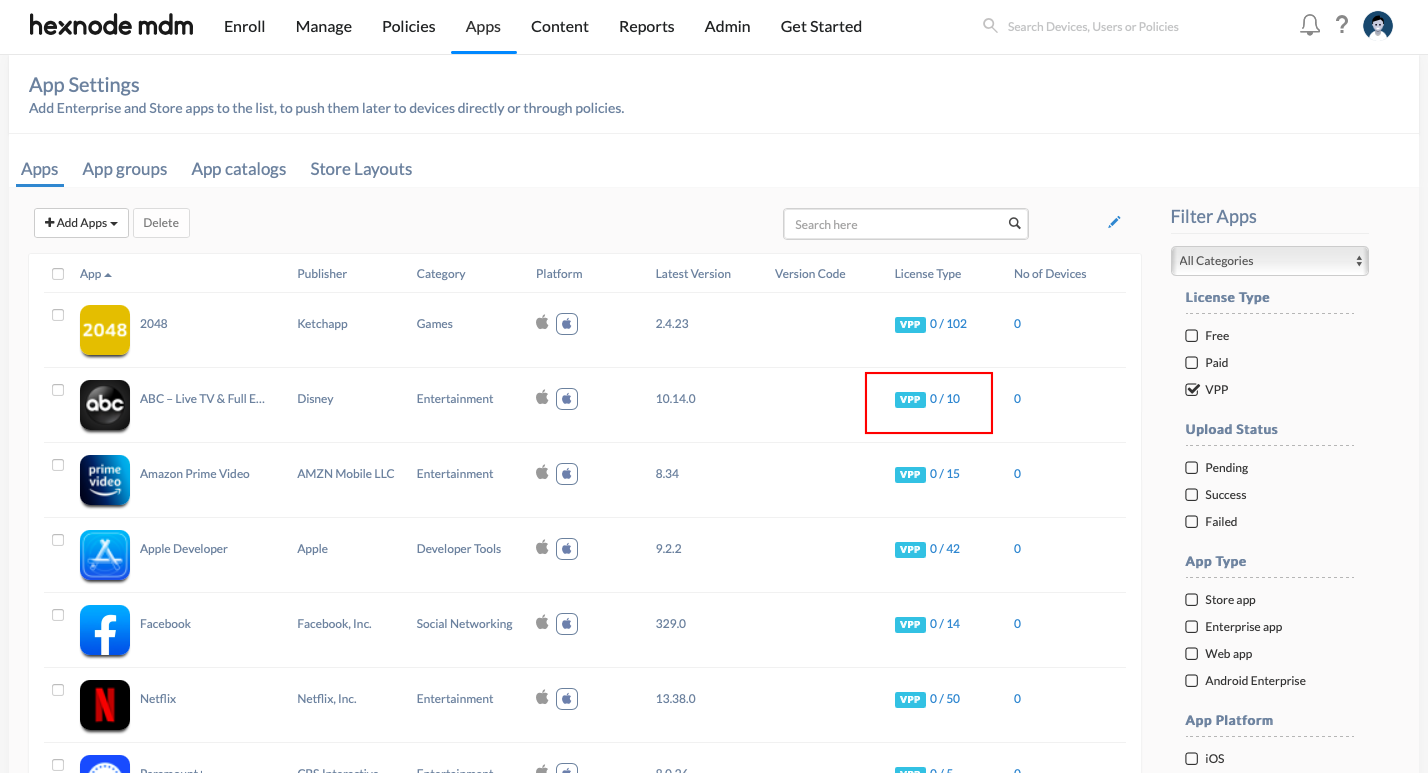The image showcases a user interface on a white background with black text headers. Prominently displayed is the title "XnodeMDM" in bold, darker black text. Adjacent to this title, there is lighter black text listing various functions: "Enroll," "Managed Policies," "Apps," "Content," "Reports," "Admin," and "Get Started." Below the "Admin" section, a blue bar highlights its selection.

To the right, a search box invites users to "Search Devices, Users, or Policies" in gray placeholder text. Alongside, there are three icons: a notification bell, a question mark for help, and a profile picture featuring a cartoon character.

On the left side, gray text reads "App Settings," followed by an instruction to "Add Experience and Store Apps to the list to push them later to devices directly through Policies." Below this, the interface is divided into sections: "Apps," underlined in blue to denote the active tab, followed by links to "App Groups," "App Catalogs," and "Store Layouts."

The interface includes a gray navigation panel with an "Add Apps" button and a "Delete" button, along with a search functionality. Further to the right, the phrase "Filter Apps" appears in gray.

Descending the right-hand panel, multiple filter categories are available: "All Categories," "License" segmented into "Free," "Paid," and "VPP" (which is selected), and "Upload Status" with options for "Pending," "Success," and "Failed." Additional filters include "App Status" (divided into "Store App," "Enterprise App," "Web App"), "Android Experience," and "iOS."

The left panel lists various application names such as "2048," "ABC Live," "Amazon Prime," "App Developer," "Facebook," and "Netflix," indicating that this interface is used for managing app deployment and organization.